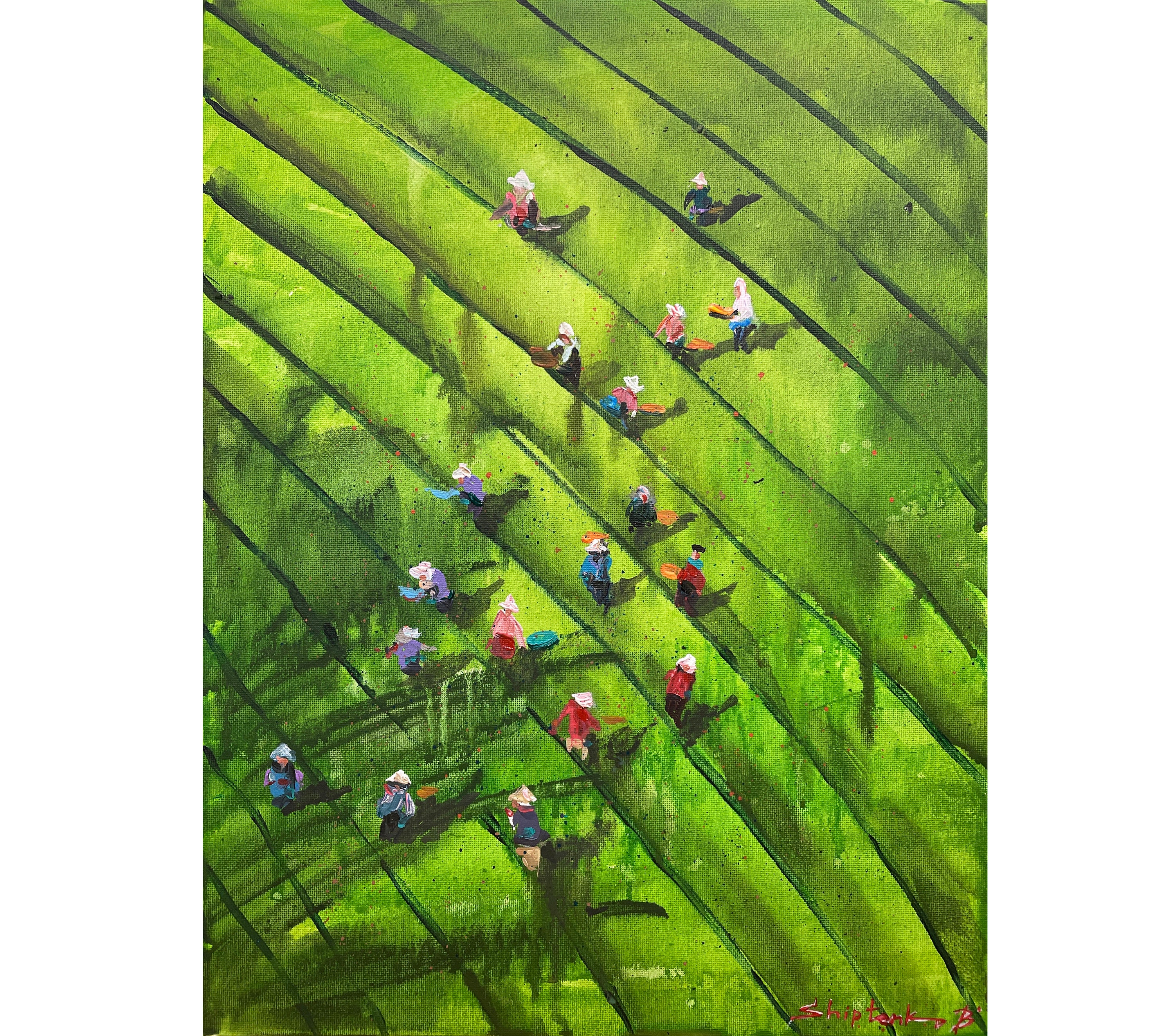This image is a vertically oriented painting that depicts an aerial view of individuals working in a rice field, rendered with pastel-like materials. The scene features diagonal, slightly curved darker lines that cut across the field, likely representing the sections of the rice paddies. The background is a light yellow-green wash, with areas of color dripping towards the bottom. Scattered throughout these green lines of the field, there are 18 individuals, depicted as small splotches of red, blue, purple, and green, all donning conical white hats characteristic of rice farmers. Some figures are sitting, while others are standing or carrying baskets, engrossed in their harvesting activities. The majority of the people are concentrated towards the bottom left-hand side of the painting, becoming fewer as they move towards the center. The artwork is signed in red lettering at the bottom right corner, although the exact signature is not clearly legible.